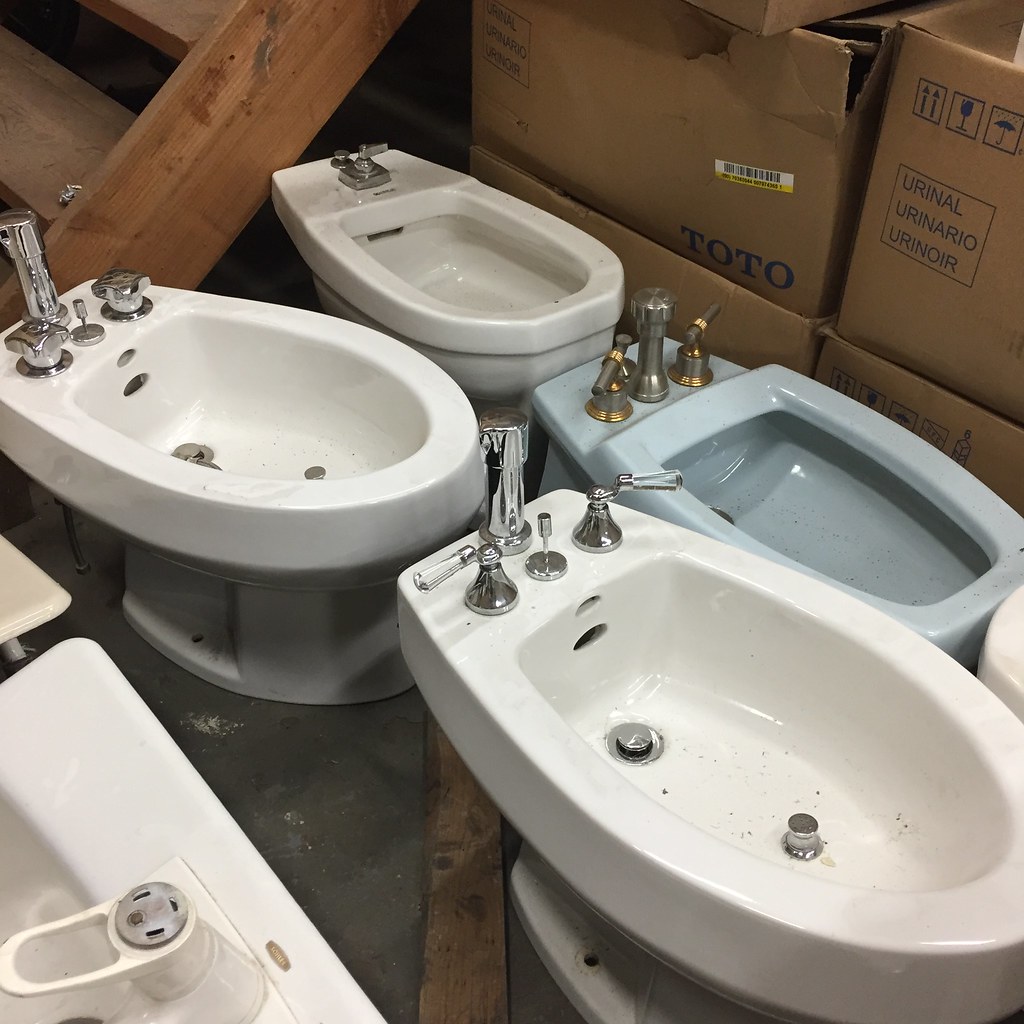The image depicts a cluttered basement-like storage area with simple wooden stairs and a cement floor, scattered with cardboard boxes. Prominently, it features four bidets: three are white porcelain, while the fourth is a distinctive baby blue with goldish handles; the others have silver handles. The bidets are arranged in varying states of cleanliness—some are notably dingy and yellowed, with black spots dotting their surfaces. They present a conundrum with their cross-like appearance between sinks and urinals, lacking traditional spigots but featuring push buttons for flushing and metal implements in their bowls. The boxes, some of which are torn open, bear the logo "Toto" and are labeled with the words "urinal," "urinario," and "urinol." The setting appears to be either a warehouse for used bathroom furnishings or a makeshift storage space, marked by its mixed flooring and the unkempt condition of the items.